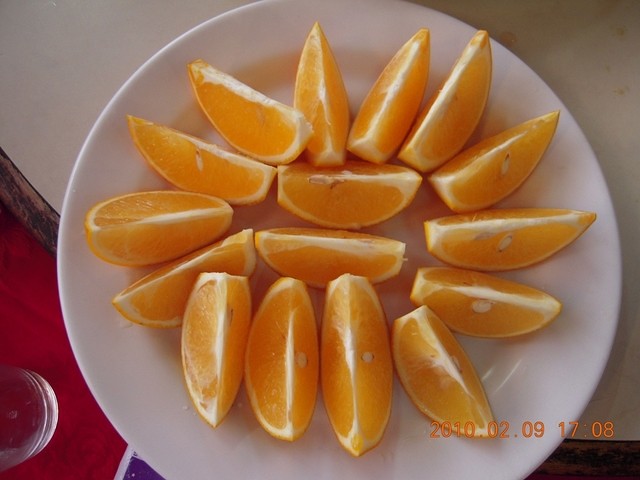The image depicts a detailed color photograph of a plain white circular plate with a slightly elevated rim, placed on the edge of a light-colored laminate counter with wood trim. Upon the plate are uniformly cut orange wedges, with some exhibiting visible seeds. Each wedge retains its peel, and the wedges are arranged meticulously, with two in the center and approximately sixteen others forming a sunflower-like pattern around them. In the lower right-hand corner of the photo, in orange letters, is a timestamp reading "2010-02-09 17:08." To the left of the plate, a clear glass of water is visible. The plate and its contents are the main focus, with no people or animals present in the scene.